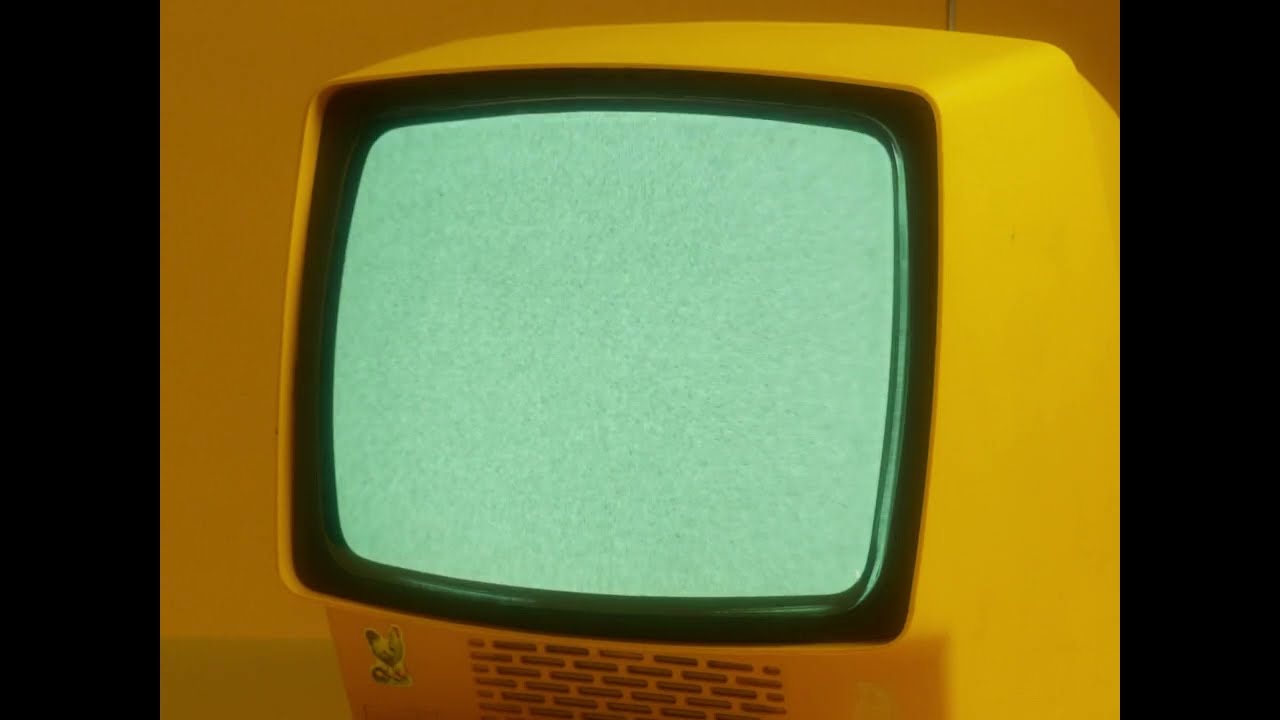The image depicts a vintage television set with a boxy, yellow frame set against a black background, extending to the far left and right edges. The center of the TV screen displays classic static — a mix of black, white, and light green specks, reminiscent of an old TV without a signal. The television's top right corner hints at a small, gray antenna, though it's mostly cropped out of the frame. Below the screen, black text is visible on the yellow casing, beside an apparent speaker area characterized by vertical slits intended for sound output. On the bottom left of the TV frame, a small sticker featuring a kitten adds a touch of charm to the otherwise utilitarian design. Overall, the TV's vibrant yellow contrasts with the darker, almost gold-yellow background that envelops the entire scene.